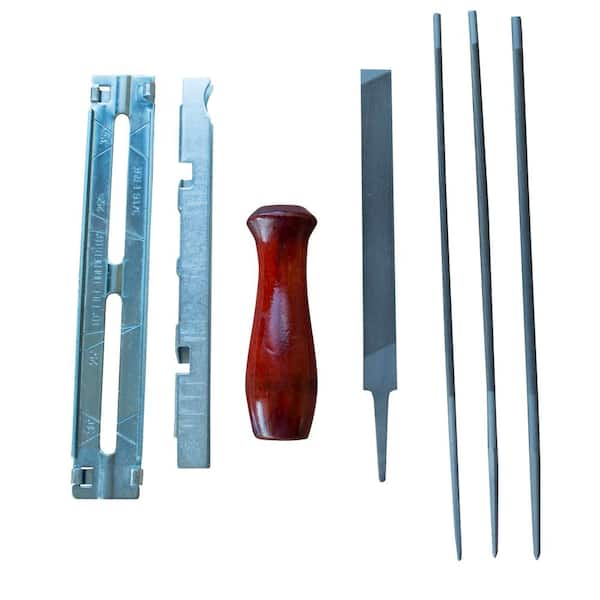This image captures a collection of metal tools and a distinctive wooden handle, meticulously arranged against a clean white background. Dominating the center of the photograph is a shiny, reddish-brown wooden handle designed for a better grip. To the left of this handle are two silver-gray metal strips resembling blades; the closest one is smaller with a central cutout, while the one further left is larger and features notches. To the right of the handle, the lineup begins with a wide flat file, followed by three long, narrow, round files—perfect for accessing and filing tight spaces. The variety and arrangement of these tools, all with similar metallic silver, gray, and white hues, highlight their intended use and functionality, possibly for precision work in wood, metal, or plastic.